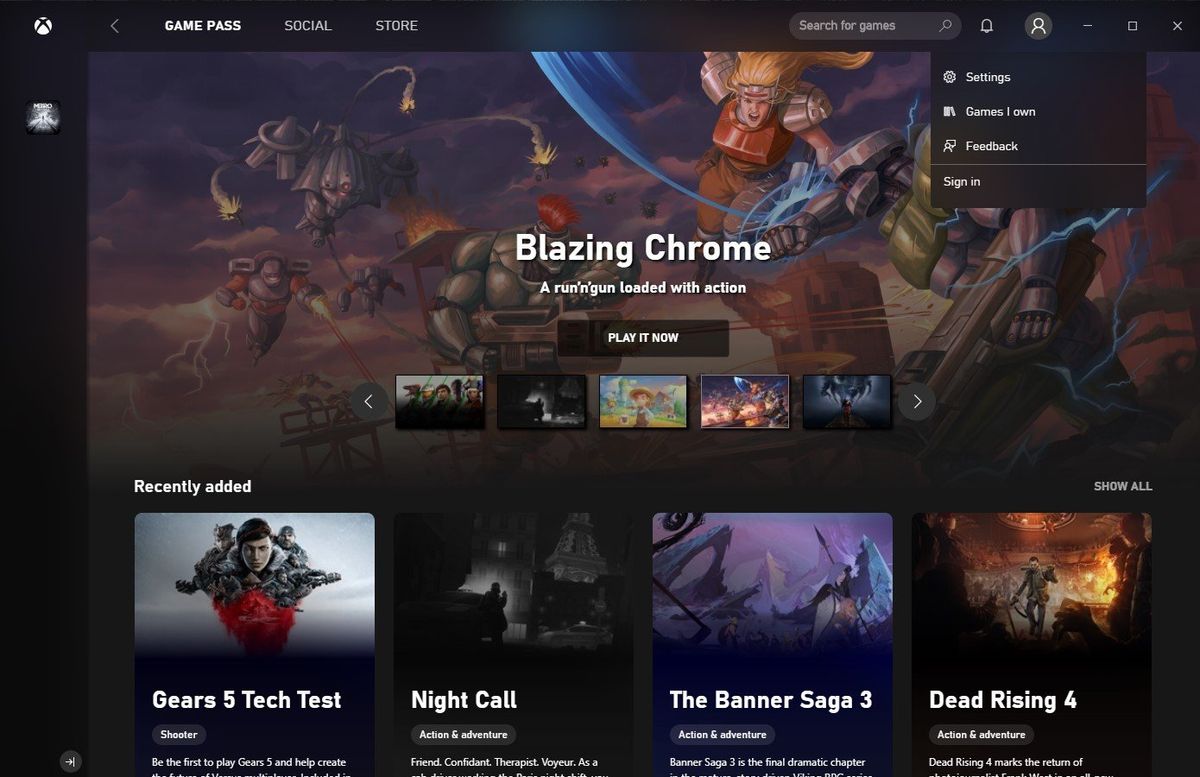Screenshot of Xbox Game Pass Interface

The image is a screenshot of the Xbox Game Pass interface, a part of the Xbox gaming platform. At the top of the screen, you can see prominent tabs labeled "Game Pass," "Social," and "Store." A search bar is available for finding games, alongside a user icon, a notification bell, and window control buttons for closing, minimizing, and maximizing the window. Currently, a drop-down menu is deployed, displaying options such as "Settings," "Games I Own," "Feedback," and "Sign In."

On the left side of the interface, there is an icon representing a game. The main area prominently features the game "Blazing Chrome," described as a run-and-gun action game. It invites users to "Play Now." Below this main feature, there are five screenshots or icons of various other games.

Towards the bottom of the screen, the "Recently Added" section showcases a few new titles. This includes:
- "Gears 5 Tech Test," a shooter game,
- "Night Call," categorized under action and adventure,
- "The Banner Saga 3," also labeled as action and adventure,
- "Dead Rising 4," another action and adventure game.

Each of these games displays relevant artwork or screenshots, although some text beneath them is cut off at the bottom of the screenshot.

The general background of the interface is dark grey. The featured "Blazing Chrome" game shows a vibrant cartoon-style scene with characters flying and shooting lasers from their hands. The image is rich with colors and characters but gradually fades into grey towards the bottom.